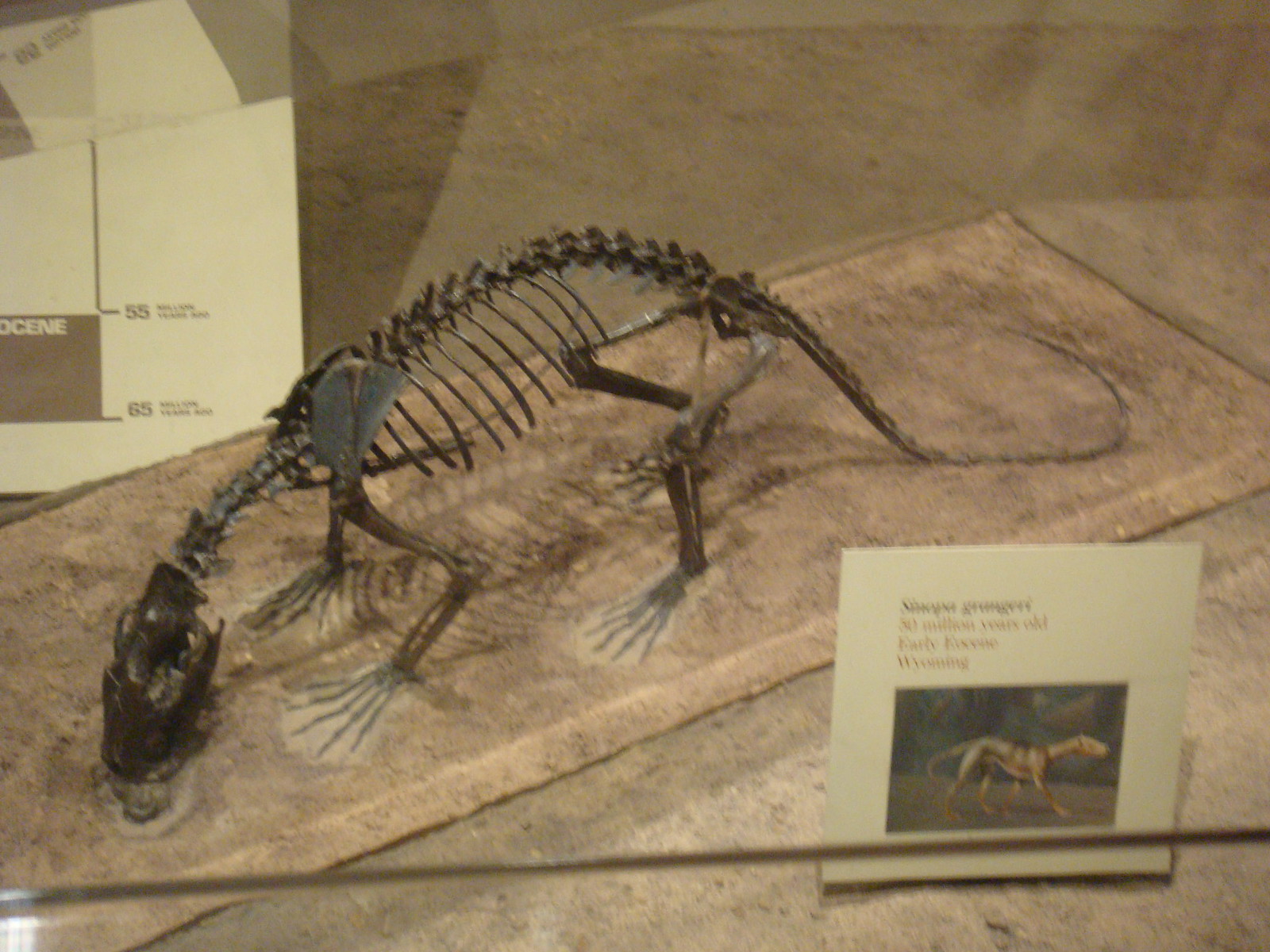The photograph captures a museum exhibit featuring a well-preserved fossil of a four-legged, dog-like creature with a long tail. The fossil is meticulously assembled to simulate its original, standing posture. Positioned on a pinkish-brown, sandy stone base, both the fossil and its platform echo the earthy hues beneath them. In front of the fossil stands a white placard with an artist’s rendition of what the creature might have looked like in life. The text on the placard is unreadable due to the photograph's blurriness, though it mentions "Wyoming" and a rough estimate of "30 million years old." The creature’s head is directed towards the bottom left corner of the image, while its tail extends upwards to the top right. The exhibit is bathed in adequate lighting, clearly showcasing the sole object in the frame amidst a well-defined museum setting.